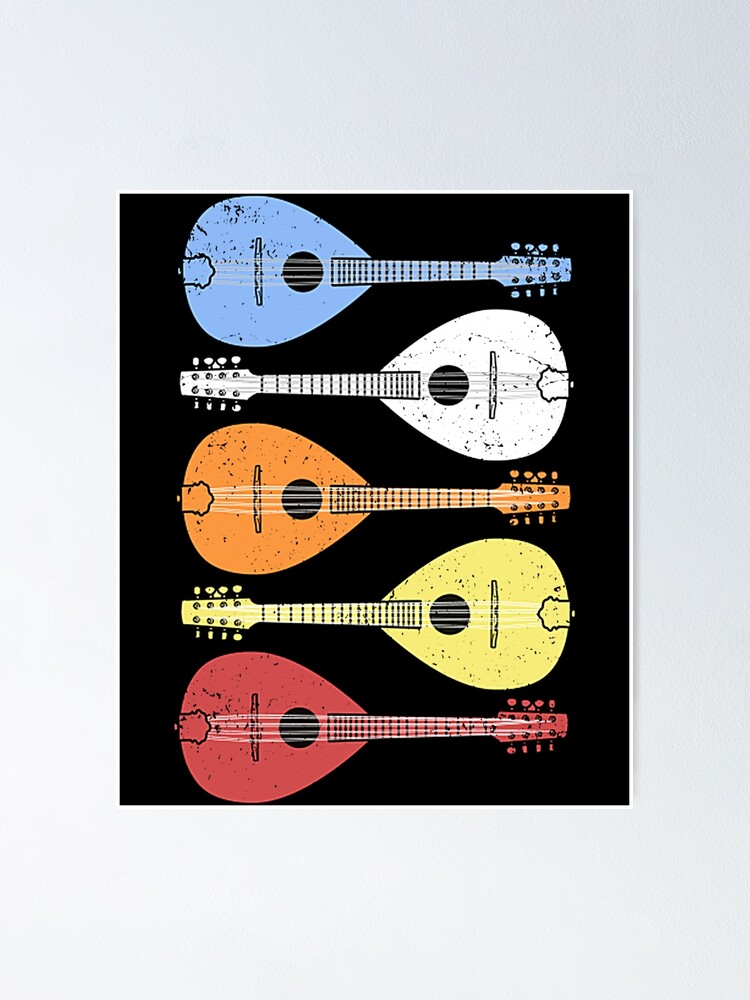This image depicts an artistic rendering of a poster, featuring a striking arrangement of five ukulele-style guitars laying sideways on a black background. Each guitar is meticulously colored: light blue at the top, followed by white, orange, yellow, and red at the bottom. The guitars are positioned alternately, with the head and body facing in opposite directions—left for blue, right for white, left for orange, right for yellow, and left for red. The entire bodies of the guitars, including their heads, share their respective colors. Their strings are uniformly white across all instruments, adding a subtle contrast to the vibrant hues. The background is dark, providing a stark contrast that makes the colors pop vividly. The design potentially serves as a poster or a magazine cover, enhancing its visual appeal with a symmetrical and orderly display, reminiscent of small fat-bodied guitars or mandolins, engaging the viewer with its harmonious color coordination and neat arrangement.